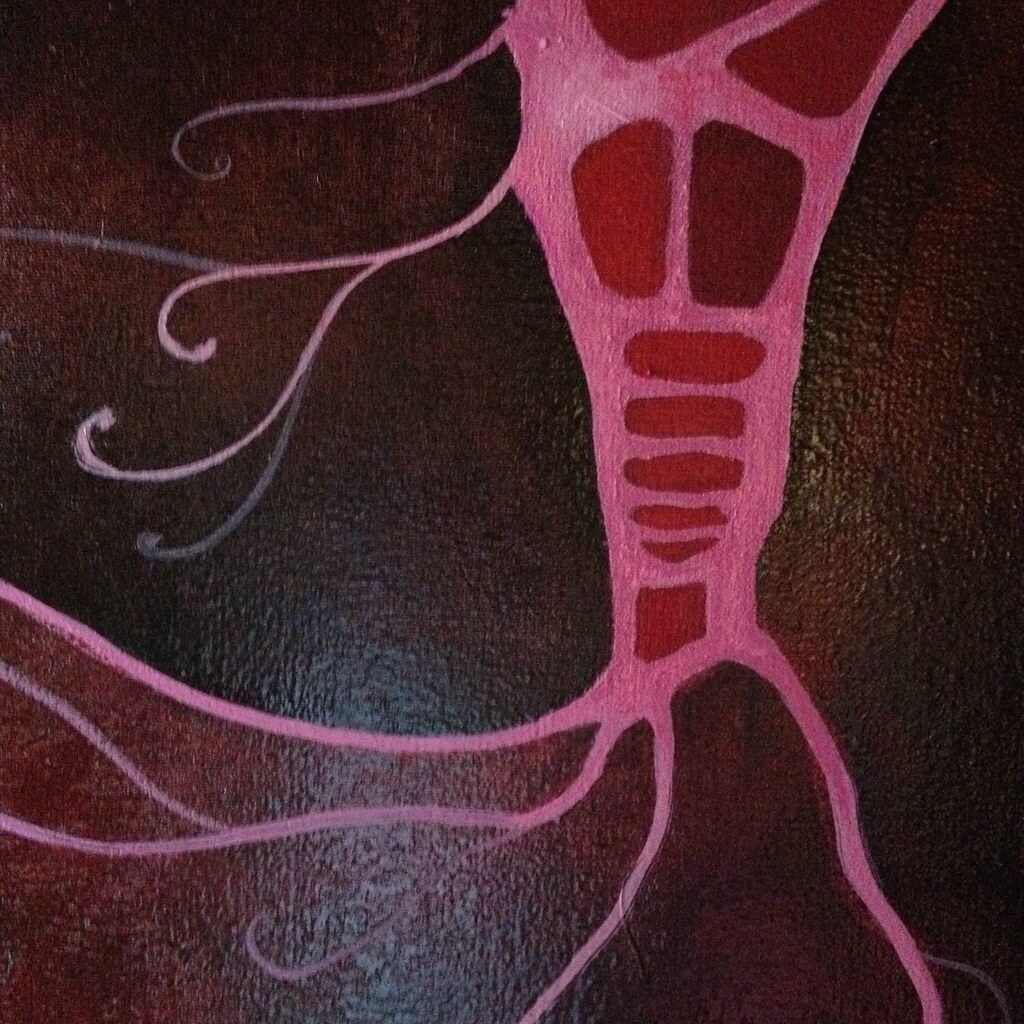This image captures an abstract painting on a dark red, almost maroon background with hints of black. Dominating the composition is a striking pink form, which resembles the shape of a Hydra organism with an upper body and tentacle-like extensions. Pink stripes weave through this central figure, adding dynamic movement. Intricate red circles and shapes are embedded within the pink structure, with one darker red shape standing out among the rest. The painting reveals a subtle glow, where light reflects off its surface, enhancing its texture and depth. Notably, the image, which is nearly square in shape, shows that the painting is unsigned.